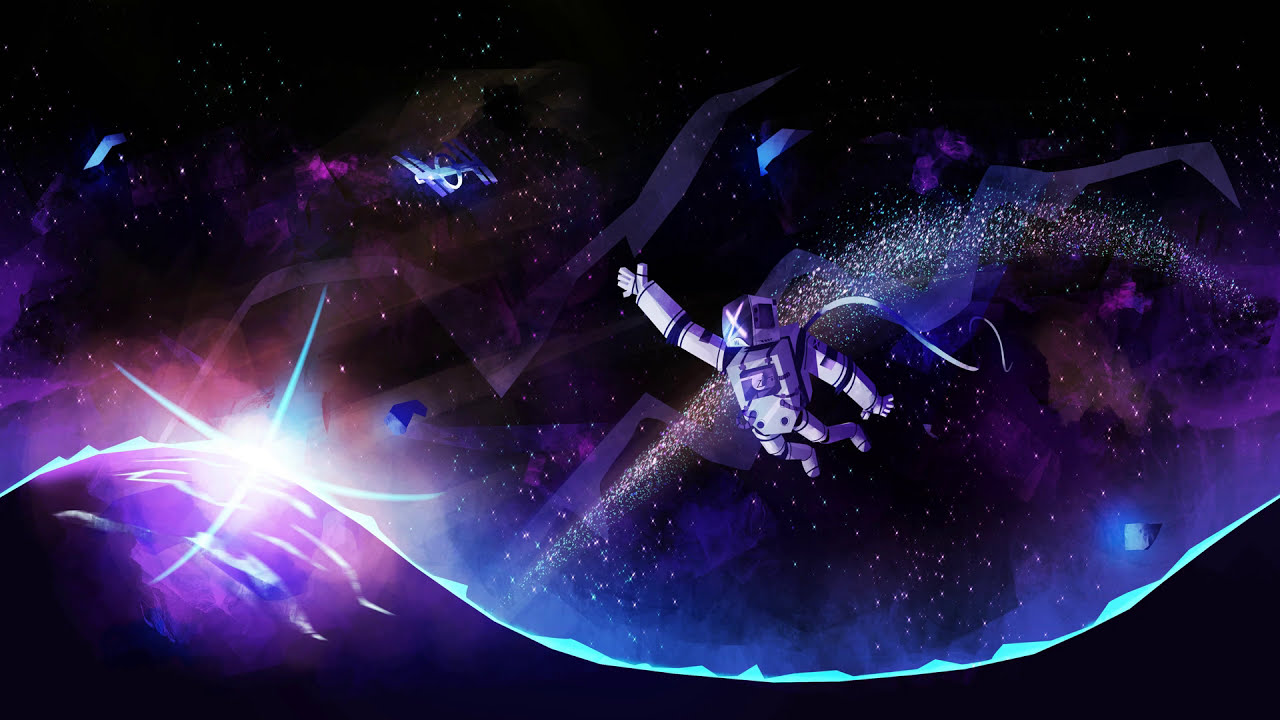The image is an animated drawing of a robotic astronaut flying through a vast, purple and blue-hued space. The astronaut has a square-shaped head emblazoned with an X, and a metallic, squarish body. Trailing behind the astronaut is a line of stars forming an arch, with the left side of the arch longer than the right. To the top left of the astronaut, there is a telescope with a circular ring in the middle. Below the astronaut is an S-shaped curve with highlighted edges, suggestive of a planetary surface, accompanied by a purplish aura. In the bottom right, there is a blue, half-arched area amidst the predominantly black background. The scene includes various stars and galaxies, along with geometric patterns and an ambiguous structure extending across the scene, adding further depth to this cosmic illustration.